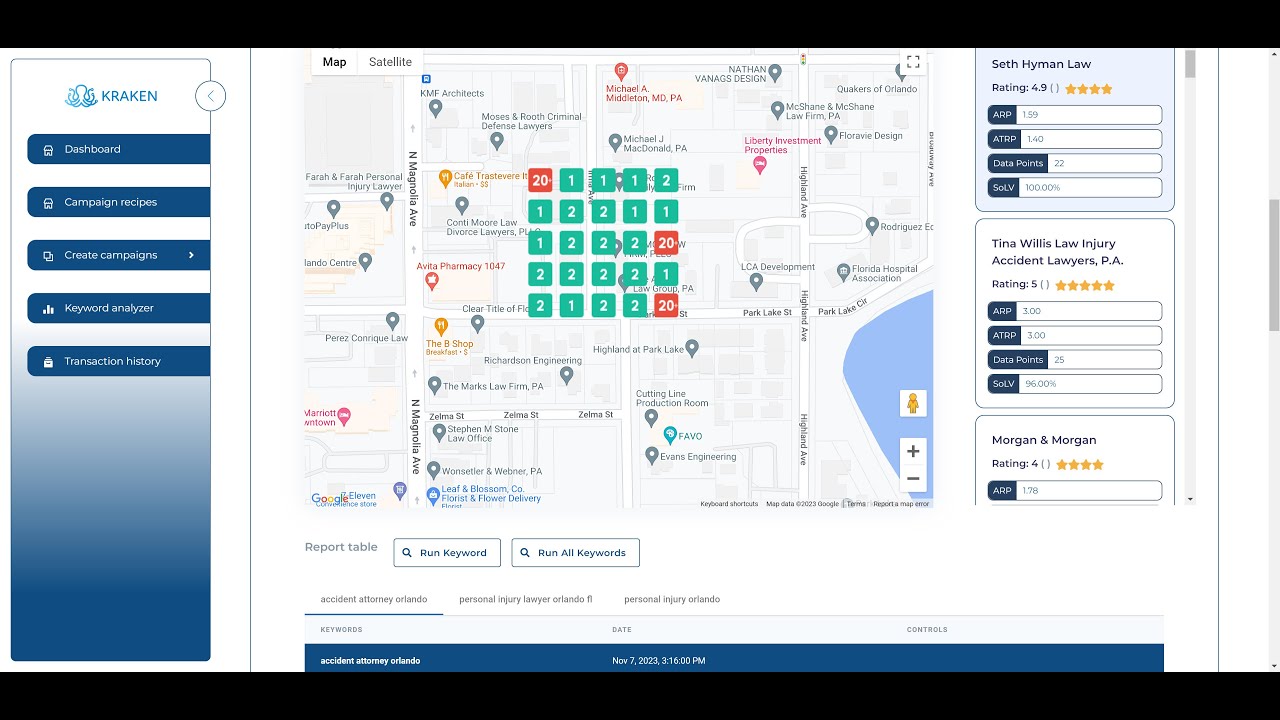The image depicts a website interface with a detailed layout. The webpage is framed by black borders on the top and bottom, and the main content sits on a white background. On the left side, there's a navigation panel that transitions from white at the top to a darker blue at the bottom. This panel includes several labeled banners for navigation options: "Dashboard," "Campaign Recipes," "Create Campaigns" (which has a right arrow indicating a submenu), "Keyboard Analyzer," and "Transaction History." 

To the right of this panel is a section featuring a grid map overlaid with small squares. The first square is red with the number 20 inside it. The following four squares are green; the first three have the number 1 and the fourth has the number 2. Subsequent lines of squares show a mix of green and red squares with numbers inside: one line shows green squares displaying 1, 2, 2, 1, 1; another has green squares with 1, 2, 2, 2, followed by a red square numbered 20. Further rows predominantly feature green squares with occasional red ones, consistently labeled with 1s and 2s.

At the bottom of the webpage, there is a section labeled "Report Table," accompanied by a search box and two buttons: "Run Keyword" and "Run All Keywords."